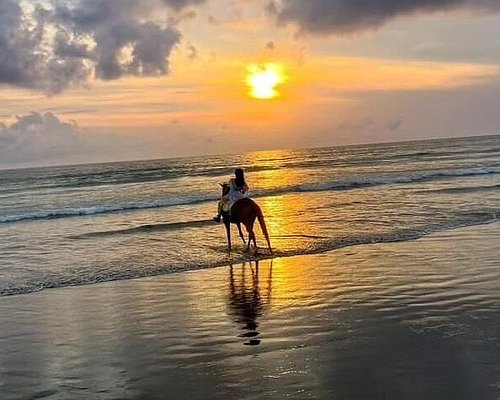A tranquil scene captures a young woman with long brown hair astride a brown horse, wading in the shallow, gentle waves of the ocean during sunset. The bottom half of the image showcases the calming, rhythmic movement of the waves, only a few inches high, cooling the horse's feet. Above, the sky is a canvas of vibrant colors—shades of yellow, orange, and pink blend beautifully against partly cloudy skies. The setting sun, slightly misshapen by clouds, casts an orange glow across the water. The horse and rider, viewed from behind, are outlined by the sunlit horizon, creating a serene reflection on the water that mirrors the graceful interplay of light and color.